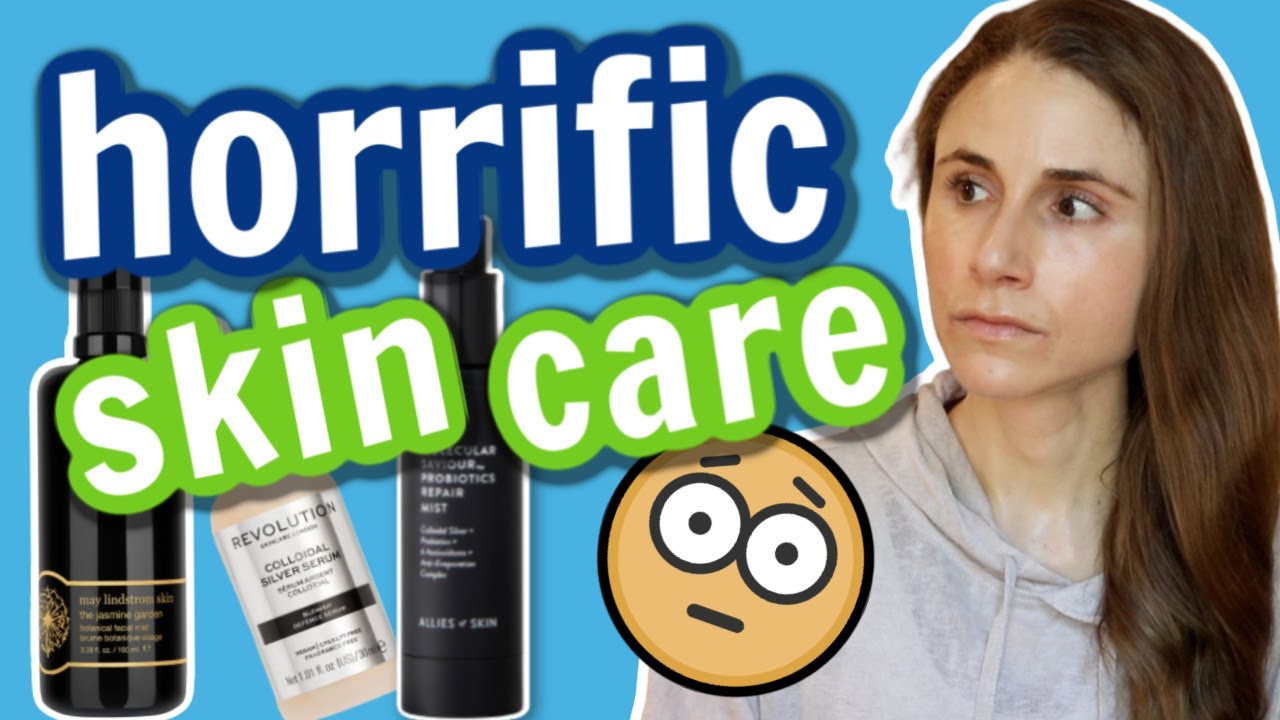In this striking image, a young woman with long brown hair, dressed in a gray hoodie, stands on the right side, looking concernedly towards the left. Dominating the left side and extending to the center is large text that reads "Horrific Skincare," with the word "horrific" in white text bordered by dark blue and "skincare" in white shaded by green. The background is a soothing blue, contrasting sharply with the troubled theme. A yellow, scared-looking smiley face with bulging eyes is positioned in the center, adding a sense of urgency and alarm. Directly below the text are three skincare products: two black bottles flanking a beige container labeled "Revolution," arranged side by side. The overall theme suggests a cautionary message about the perils of using certain skincare products, potentially making this an impactful YouTube thumbnail aimed at educating viewers on products to avoid.